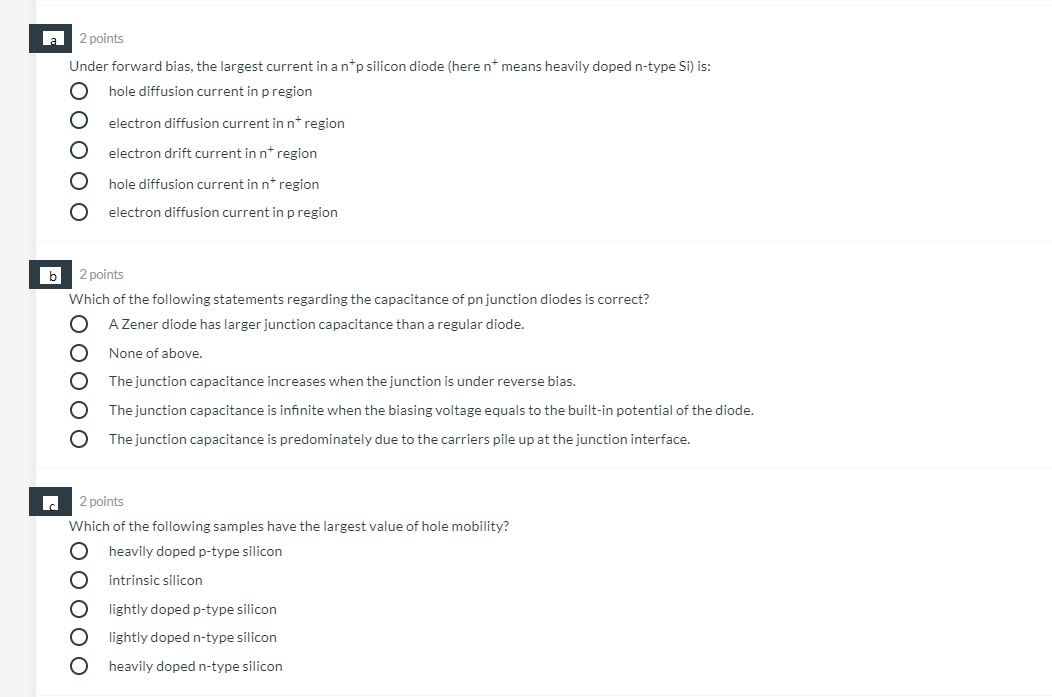The image features a multiple-choice test displayed on a white background. On the left side, there is a vertical gray bar. The first question, marked by a bold black letter "A" followed by a lowercase "a," indicates that it is worth two points, shown in light gray text. The question reads, "For biasing the largest current in a heavily doped p-type silicon diode, what is the predominant carrier transport mechanism in region X?" Below this question, there are five answer choices, each accompanied by a circle to be selected. The answer options are:

1. Hole diffusion current in region X
2. Electron diffusion current in region X
3. Electron drift current in region X
4. Hole diffusion current in region Y
5. Various other choices

Following this section, there is a black box containing the letter "B." This section is also worth two points and poses the question, "Which of the following statements regarding [a specific topic] is correct?" Beneath this question, five potential answers are listed, each with a selection circle next to it.

In the third section, another black box marked with the letter "C" appears. This question, also worth two points, asks, "Which of the following samples has the largest value of hole mobility?" Similar to the previous questions, five different answers are provided, each with a corresponding circle for selection.